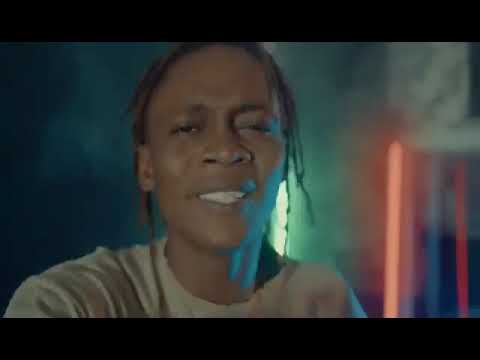The image portrays a youthful African-American man, likely in his late teens or very early twenties, with closely cropped, narrow dreadlocks that fall loosely around his head and ears. He has medium brown skin and faint eyebrows. The man is either smiling or mid-conversation, as his teeth are visible. He is wearing a white t-shirt and is seated in an interior setting. Behind him, to the left, a window is partially visible, while the wall features a dark grayish-green hue. On the right side of the image, a railing highlighted in a red glow stands out among other colorful, fluorescent lights, suggesting a vibrant background. The setting appears to be dimly lit, possibly at night, giving the overall scene a darker ambiance. The photograph is slightly blurry but still discernable.